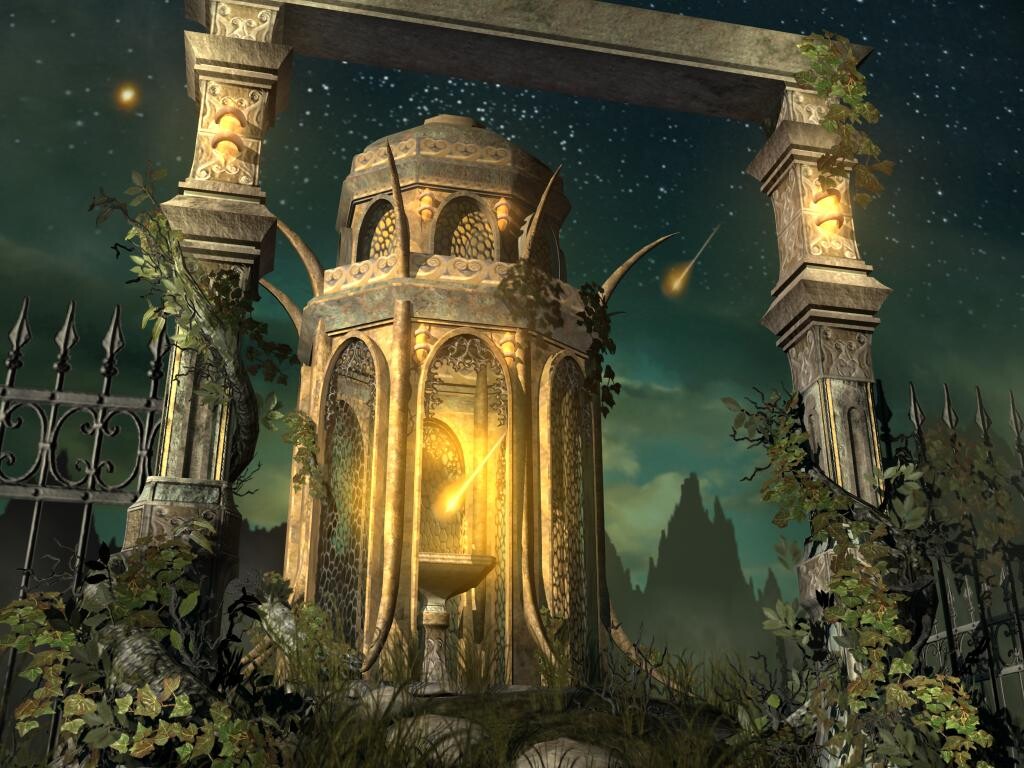The image portrays an animated, video game-like scene taken at night, featuring a grand, illuminated cement structure reminiscent of ancient architecture. This intricate structure, set within an octagonal base with arched openings, is surrounded by a black wrought iron fence with pointed tops. The building has a central basin or fountain and numerous pillars adorned with vines, giving it a historic ambiance. The roof of the structure includes spikes that curve outward, topped with hanging lights. The background features a dark sky with a blend of dark blue, earthy green, and black hues, filled with stars, a yellow comet, and jagged, eerie mountains. A serene yet mysterious atmosphere pervades the scene, inviting exploration and curiosity.